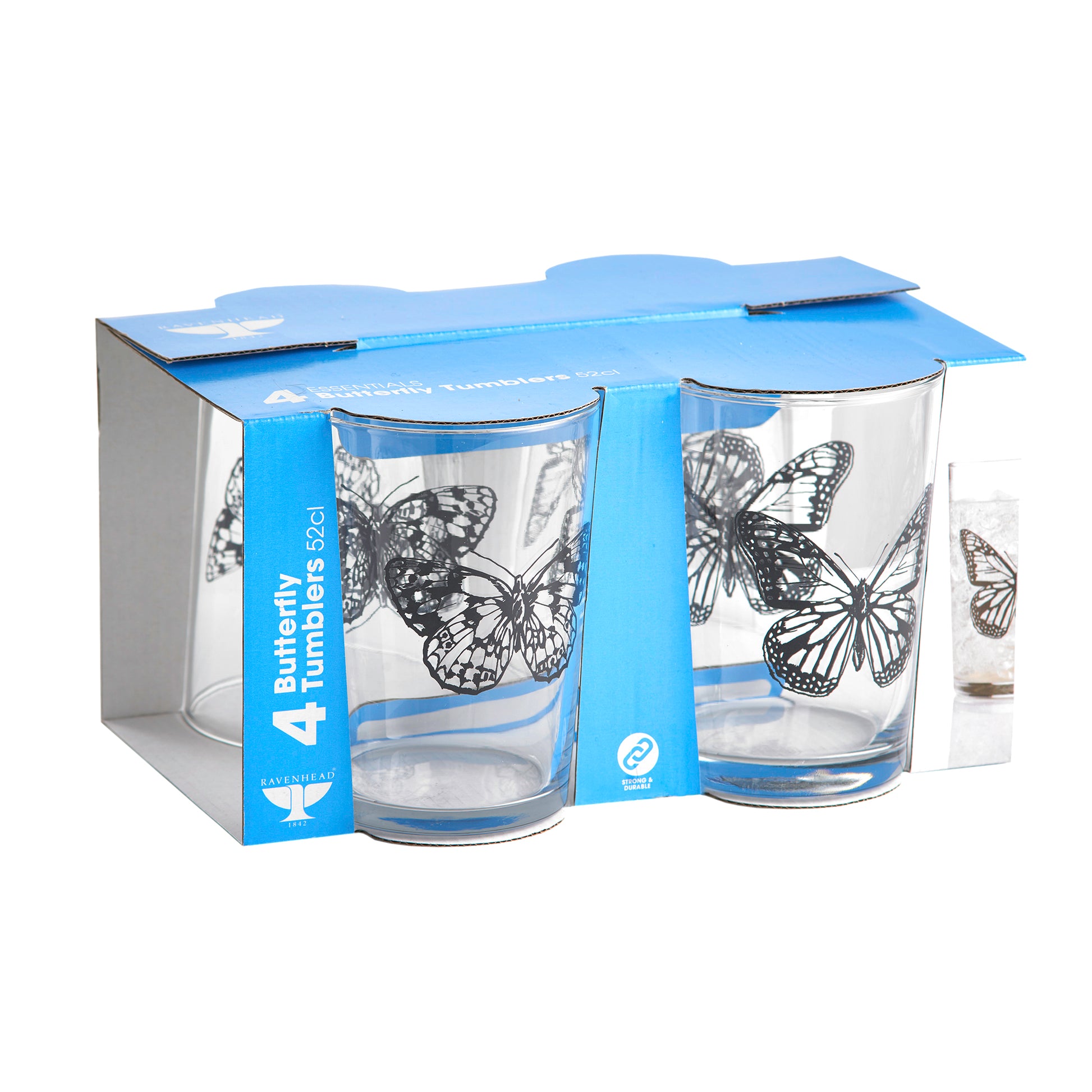This image features a carton containing four tumblers, typically found in a retail store setting. The packaging consists of a blue cardboard wrap that securely encloses the tumblers while leaving the front side partially exposed, revealing the glassware inside. The back side of the carton also allows visibility of the tumblers. Along the left side of the blue cardboard, white lettering prominently states "Four Butterfly Tumblers, 52 Centiliters" and identifies "Raven Head" as the manufacturer. The tumblers themselves are adorned with delicate butterfly designs, adding an elegant touch to their appearance.